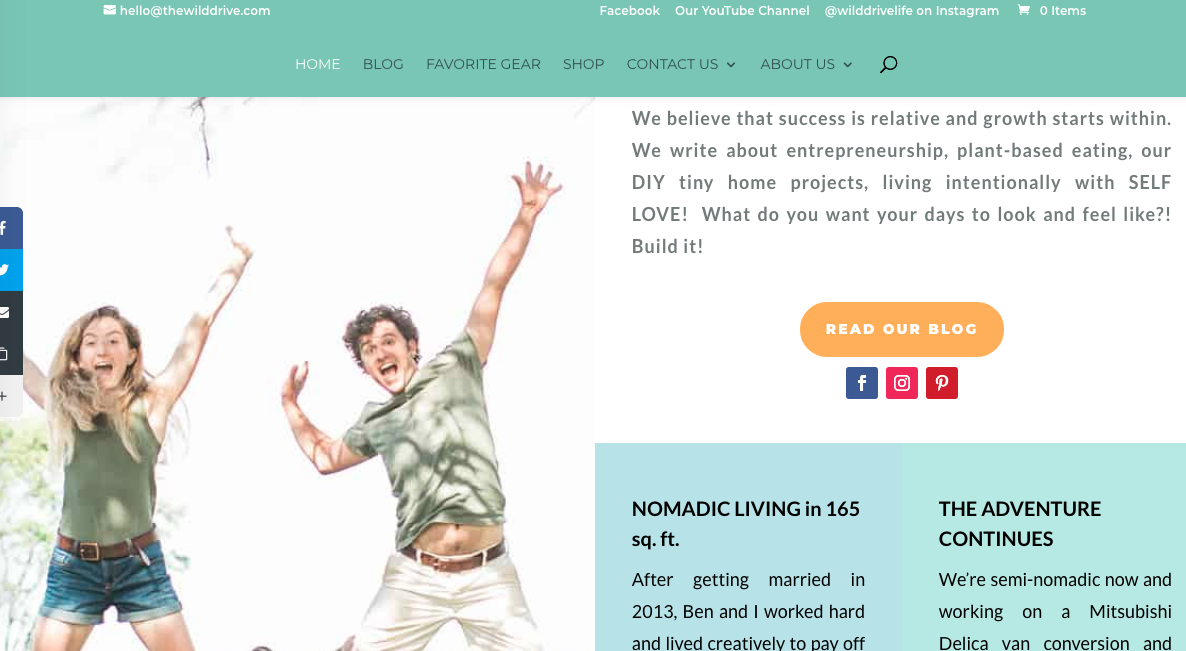**Website Screenshot Description**

The screenshot captures the homepage of a website with a teal-colored banner at the top. In the top-left corner, there's an email icon accompanied by the email address "hello@thewilddrive.com." The top section also prominently displays social media links, including Facebook, their YouTube channel, "Wild Drive Life" on Instagram, and a shopping cart icon with zero items.

Below the banner are the main navigation sections. "Home" is highlighted in white text, indicating it is the currently selected section. The other sections, displayed in black text, include "Blog," "Favorite Gear," "Shop," "Contact Us" (with a drop-down menu), "About Us" (with a drop-down menu), and a search icon.

The main content area features a vivid image on the left side of two individuals, both with either blonde or brown hair, energetically jumping with their arms raised and mouths open. They are both dressed in green shirts; the person on the left wears blue jean shorts with a brown belt, while the person on the right wears white shorts with a brown belt.

To the right of the image is motivational text: "We believe that success is relative and growth starts within. We write about entrepreneurship, plant-based eating, our DIY tiny home projects, living intentionally with self-love. What do you want your days to look and feel like? Build it." Beneath this message is a yellow button with white text that prompts visitors to "Read Our Blog," along with icons for Facebook, Instagram, and Pinterest.

Further down, a blue box is partially visible with text beginning, "Nomadic living in 165 square feet. After getting married in 2013, Ben and I worked hard and lived creatively to pay off," which then gets cut off. Adjacent to this is another box that also gets cut off, but starts with, "The adventure continues. We're semi-nomadic now and working in a Mitsubishi Delica van conversion."

This detailed description provides a clear and comprehensive view of the website's layout and content, ensuring users get an accurate sense of the site's structure and focus.